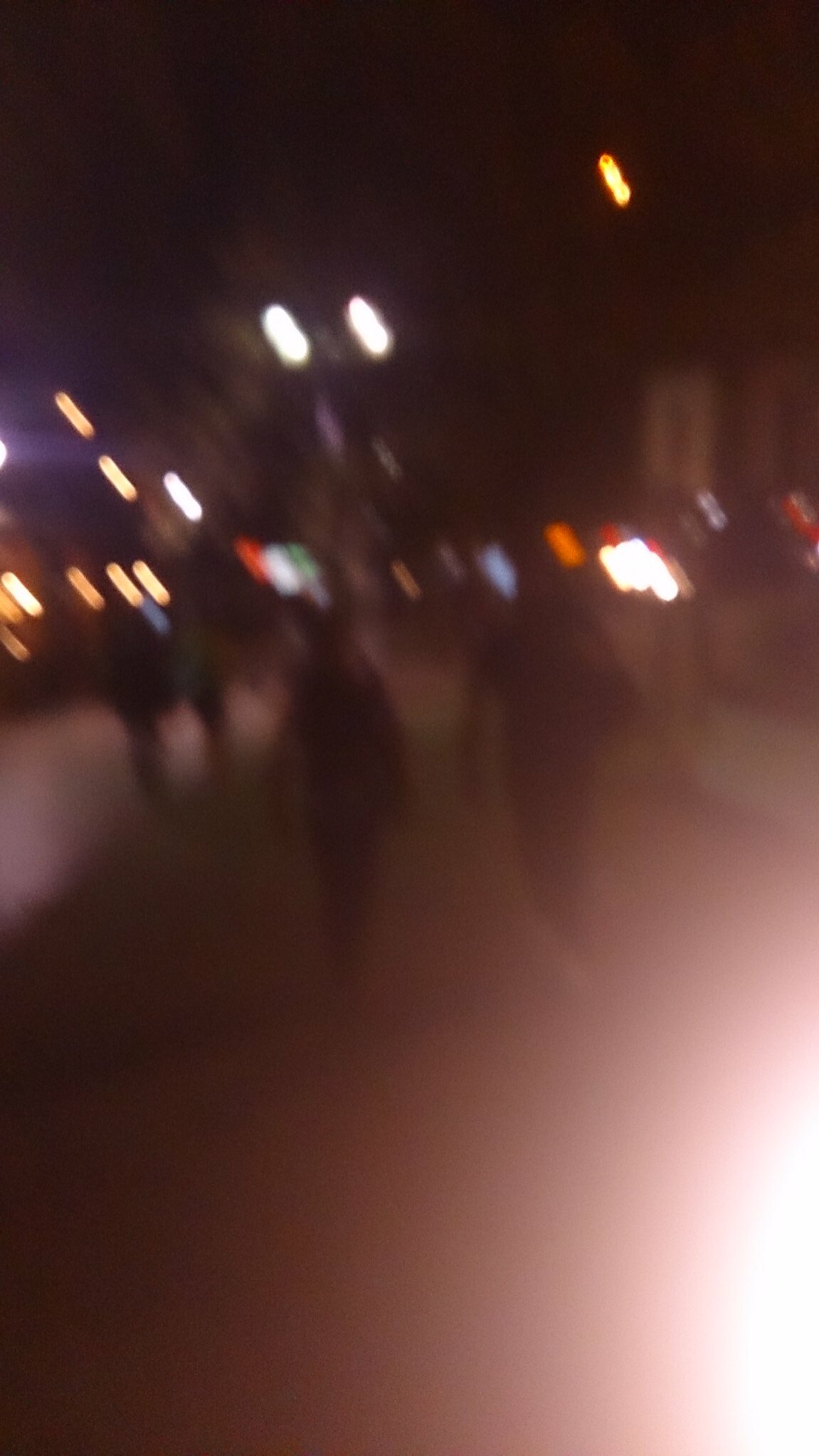In this blurry nighttime photograph taken outdoors, the scene transitions from an indigo blue to a brown-black sky as you move from left to right. Prominent streaks and blurs of lights adorn the image, showcasing varied colors including orange, white, red, and green, with some originating from street signs and car headlights. In the foreground, positioned slightly off-center to the left, are two more prominent silhouettes—potentially a taller male and a petite female—walking through what appears to be grassy terrain. Faded in the background are two additional figures towards the left side, adding depth to the scene. These silhouetted individuals seem to be heading towards a bustling downtown area, illuminated by the myriad blurred lights. The image overall is grainy and hazy, making it difficult to discern finer details or specific sources of the lights.